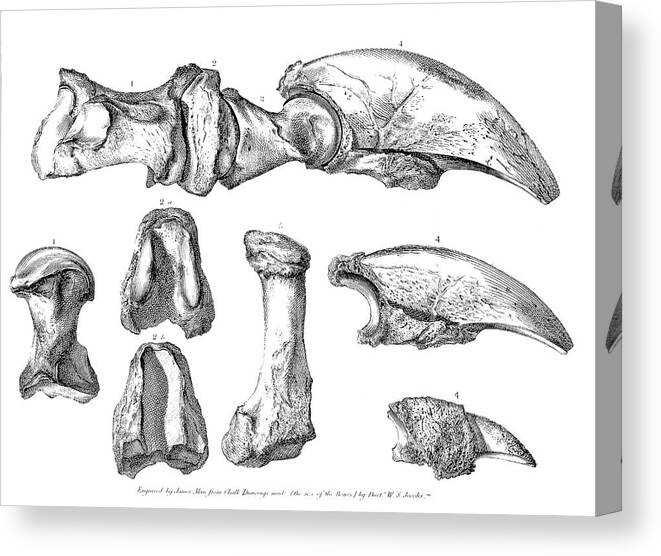The image depicts a three-dimensional, white-framed canvas featuring a black and white pencil drawing of various skeletal elements. The canvas has an intricate design that extends slightly outwards, giving it a "sticky-outy" effect. The bones, which are labeled numerically (1, 2, 3, 4, and 2A), range in appearance from long, cylindrical shapes that resemble non-human bones to shorter, round-topped and Hershey Kiss-shaped bones. Toward the right side and bottom of the frame, the design wraps around to include more skeletal images that are typically unnoticed in conventional pictures. At the very bottom of the canvas, there is a cursive legend that is too small to be legible, possibly including a signature or title that mentions being "empowered by Jesus." Overall, the artwork showcases around eight distinct bone descriptions, carefully detailed and somewhat ambiguous as to the exact species of origin.